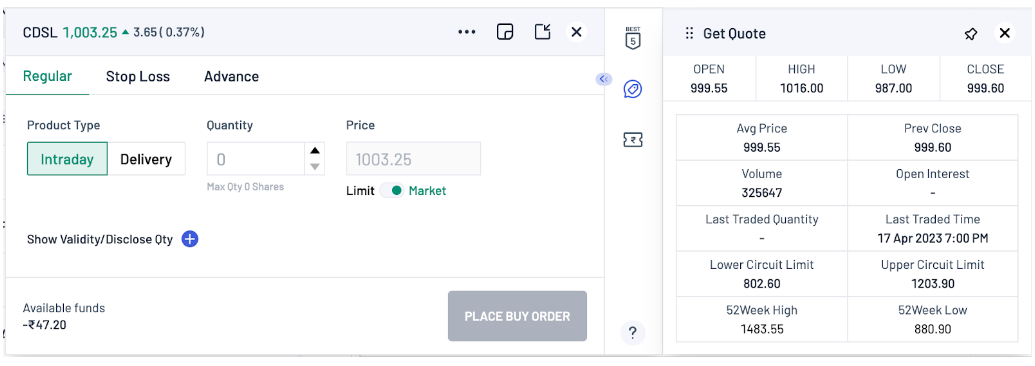The image depicts a meticulously detailed financial dashboard screen, divided into two main sections, each outlined with a gray border and further accented with a light blue border at the top.

**Left Section:**

- **Header:** 
  - The top portion features the text "CDSL" in black, followed by "1,003.25" in green.
  - Adjacent to these figures is an upward-pointing green triangle, indicating a positive change.
  - Below, in black, the figures "3.65" and "0.37%" are displayed, denoting the percentage change.
  
- **Icons and Dividers:** 
  - An ellipsis (three dots) is followed by a paper icon with a black arrow.
  - Next, a circle with a black "X" is visible.
  - A white vertical divider separates this content from the ensuing elements.
  
- **Miscellaneous:**
  - The division contains the text "Best of Five" in black.
  - A bluish text bubble shape, followed by an indistinguishable text that resembles a ticket or a "Z", then another black question mark.

**Right Section:**

- **Actionable Items:**
  - The phrase "Get Quote" in black is displayed, along with a nail icon and a white circle with an "X".
  
- **Tabs and Options:**
  - Tabs include "Recline" in green, "Stop Loss" and "Advance" in black.
  - Options are listed as "Product Type," "Quantity," "Price" in black.
  - "Intraday" in green, and "Delivery" in black.
  
- **Inputs and Pricing Details:**
  - "Quantity" shows as "0."
  - Under pricing, it lists "1,00.35" and "Limit" in black.
  - "Market" is in green.
  - Additional options include "Sold Validity/Disclosed Quantity" in black.

**Market Summary:**

- "Open: 999.55" in black.
- "High: 1016.00" in black.
- "Low: 987.00" in black.
- "Close: 999.60" in black.
- "Average Price: 999.55" in black.
- "Previous Close: 999.67" in black.
- "Volume: 3258.47" in black.
- "Open Interest" is shown as a dash.
- "Last Traded Quantity" is shown as a dash.
- "Last Traded: 17 APR 2037 PM."
- "Lower Circuit: 802.60" in black.
- "Upper Circuit Limit: 1203.90" in black.
- "52 Week High: 1483.55" in black.
- "52 Week Low: 880.90" in black.

The dashboard appears to be an interactive and comprehensive tool for monitoring financial market metrics, with clear delineations between different data sets and interactive elements for user engagement.